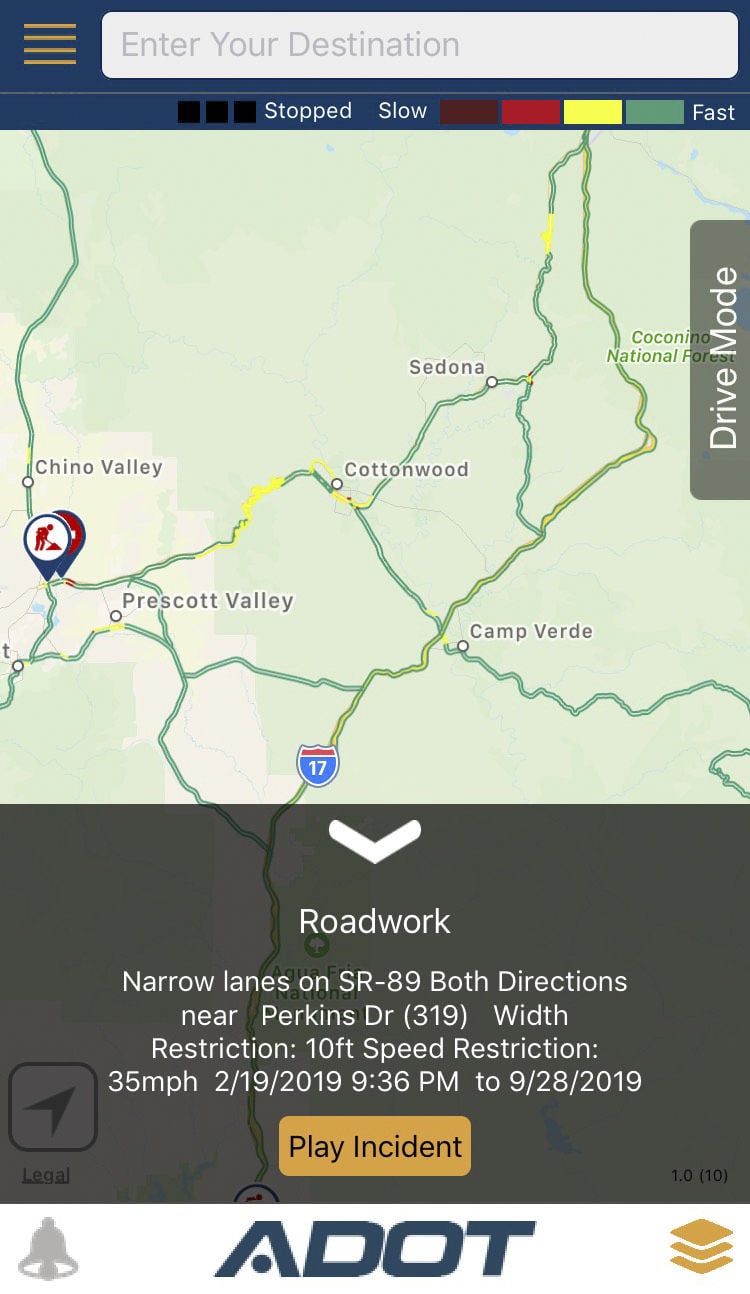Screenshot of a mobile phone displaying a navigation app. On the right side of the screen, there is a semi-transparent brown square labeled "Drive Mode." The central portion of the screen features a map with Highway 17 prominently highlighted. Several towns are indicated on the map, including Prescott Valley, Chino Valley, Cottonwood, Camp Verde, and Sedona. An alert from the Arizona Department of Transportation (ADOT) is visible at the bottom of the screen, detailing roadwork on SR 89 near Perkins Drive. The alert specifies narrow lanes in both directions with a width restriction of 10 feet and a speed restriction of 35 miles per hour, effective from February 19, 2019, at 9:36 PM to September 28, 2019.